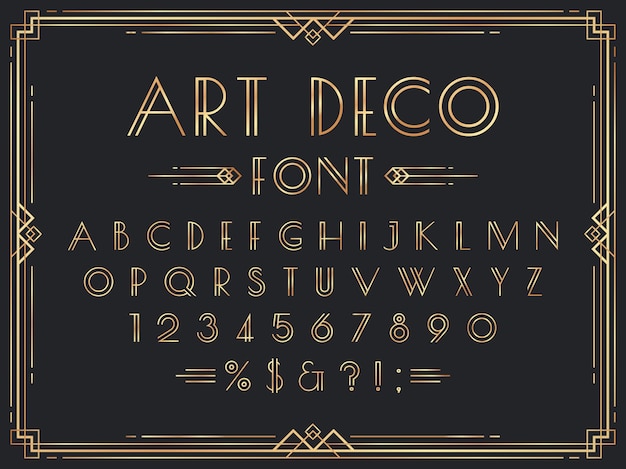The image depicts a meticulously designed modern sign with a black background and gold accents, exuding a quintessential Art Deco style. Central to the composition are the words "Art Deco Font" rendered in a striking Art Deco typeface. The font is reminiscent of the kind used in the Great Gatsby movie, characterized by geometric elegance and intricate details. The sign features the complete alphabet from A to Z, the numbers 1 through 9 followed by a 0, and various special characters including a percentage sign, dollar sign, ampersand, question mark, exclamation point, semicolon, and a colon, all in golden lettering.

The design is enriched with decorative elements: around the words "Art Deco Font" are two interconnecting diamonds and three stripes extending outwards, creating dynamic motion lines to the left and right. Encircling the entire sign is a geometric border of triangles and lines that mirrors the Art Deco aesthetic. Additionally, the corners are adorned with patterned embellishments that mimic vintage photo corners, enhancing the overall thematic cohesion. This visually captivating poster appears to be a creation designed on a computer, showcasing the timeless elegance and stylistic features of Art Deco design.